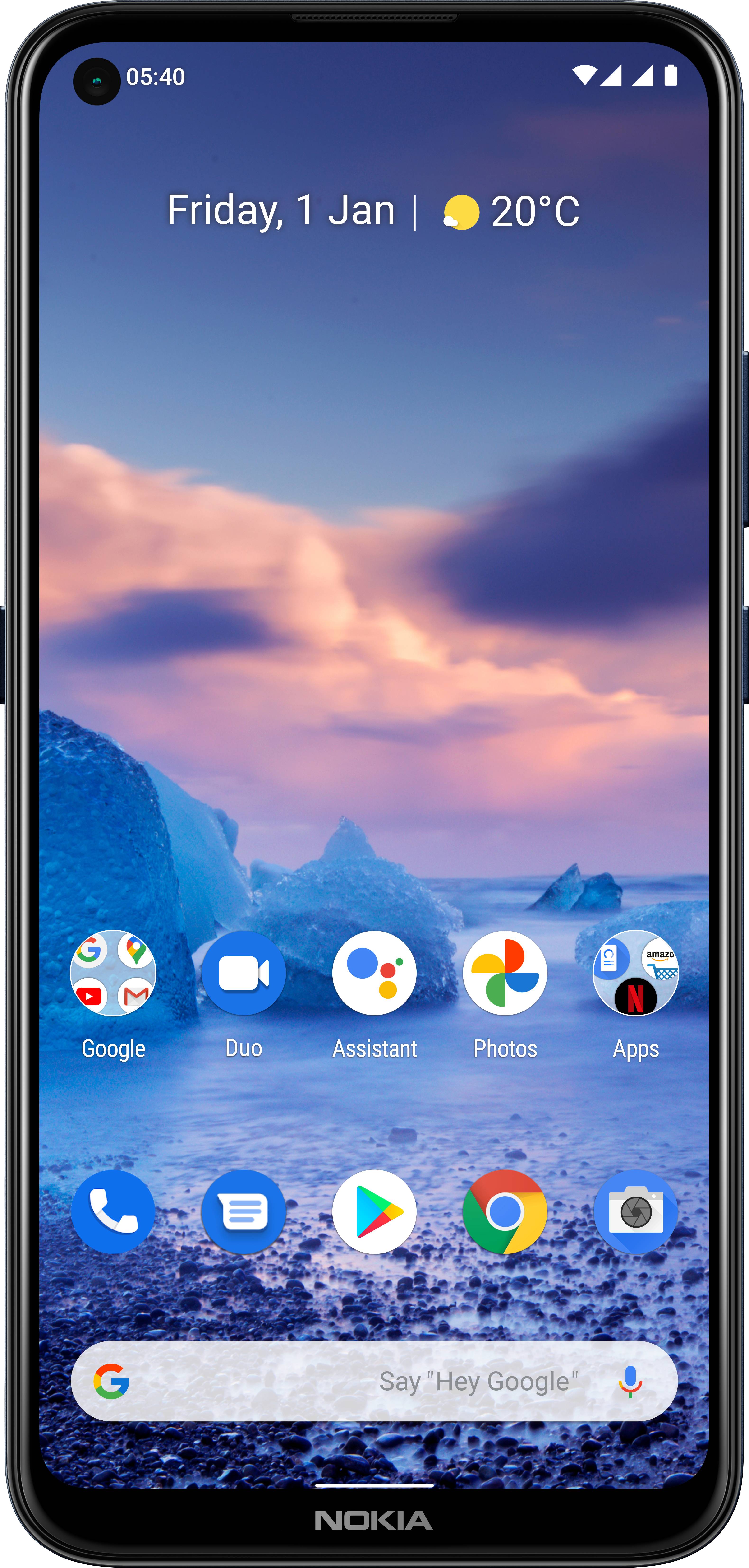This digitally rendered image features a sleek Nokia smartphone, framed with a smooth black border. The device is equipped with a single button on the upper-middle section of the left side, and two additional buttons situated towards the middle of the right side. 

The phone’s screen displays a wallpaper depicting a tranquil shoreline scene with water lapping against a rocky beach, and what appears to be icebergs floating majestically in the ocean. The distant horizon shows a blend of pinkish-purple hues, indicative of either a sunrise or sunset, with ethereal clouds enhancing the serenity of the scene. 

In the top left corner of the screen, white text displays the time as 5:40. The top right corner showcases icons for cell phone coverage, Wi-Fi connection, and battery status. Centrally positioned just below the top margin, the date is displayed as "Friday, 1 January," accompanied by a sun icon with a temperature reading of 20 degrees Celsius. 

Below the date and weather information, there are two neatly arranged rows of app icons, each row containing five apps. At the very bottom of the screen sits a Google search bar, enhancing the phone's user interface with easy access to search functionality.

Finally, the very bottom edge of the phone features the brand name "Nokia," elegantly printed in white on the black outer rim.